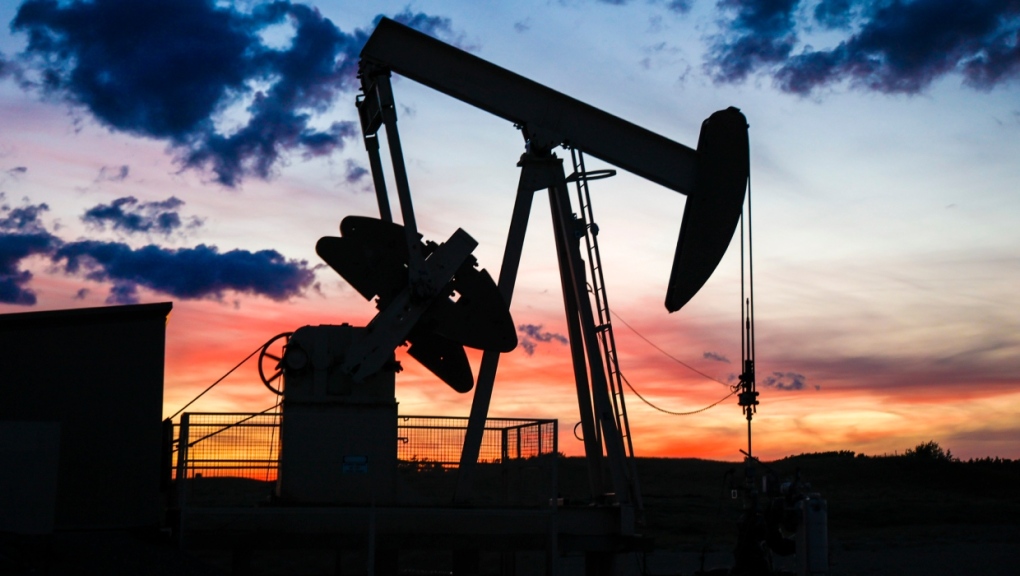This is an evocative sunset or sunrise scene featuring an oil pumpjack positioned centrally in a wide horizontal rectangular frame. The sky, splashed with vibrant hues of dark blue, light blue, orange, purple, and yellow, takes up the top three-fourths of the image, with orange-yellow clouds hovering at the horizon, suggestive of either dawn or dusk. Silhouetted against this colorful backdrop, the pumpjack stands out in stark black, its details veiled in shadow due to the low light. The pumpjack rests on triangular legs, with two parallel rods extending from the left side, each ending in a rectangular shape, hinting at the mechanical nature of the machine. A long horizontal beam stretches across the main structure, connecting to a vertical rectangle with a pointed end, from which black cables droop to the ground. At the bottom left, partially obscured in the darkness, there is the faint outline of a barrel and the side of a shed, both adding context to the scene. The ground below the silhouette is wavy and dark, indicating grassy terrain. Overall, the image captures the serene yet industrious atmosphere of an oil field at the edge of daylight.